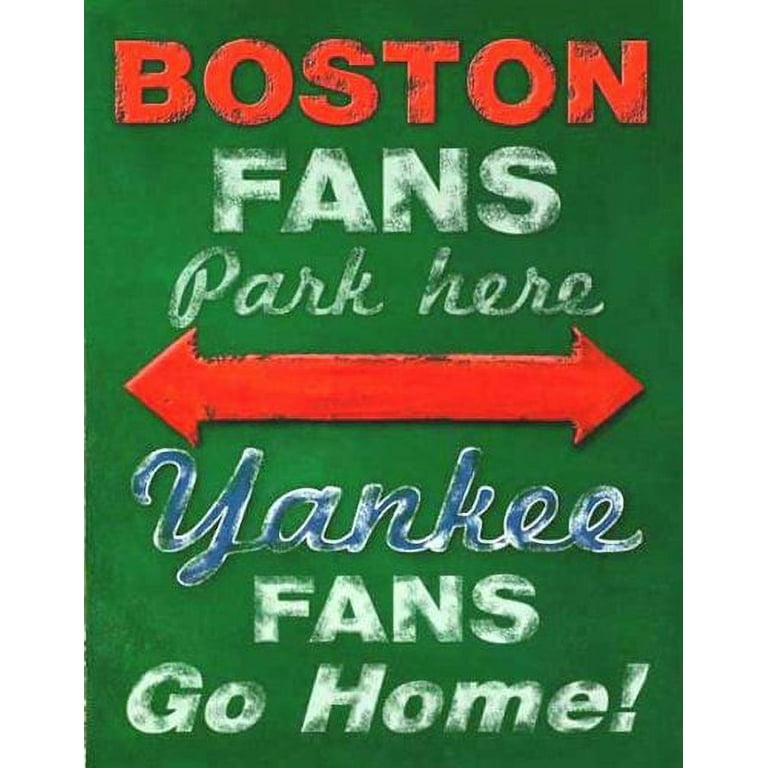This full-color poster features a dark green background with various texts in red, white, and blue. At the top, the word "Boston" is prominently displayed in bright red block letters. Directly below, in bold white letters, it reads "Fans." The text "Park Here" follows in white cursive script. A bright red double-ended arrow stretches horizontally, pointing in both directions, beneath which the text "Yankee" appears in blue cursive script. Aligning the bottom, bold white block letters declare "Fans Go Home!" punctuated with an exclamation mark. The contrasting styles and colors emphasize a clear message to visitors regarding parking preferences for Boston and Yankee fans.